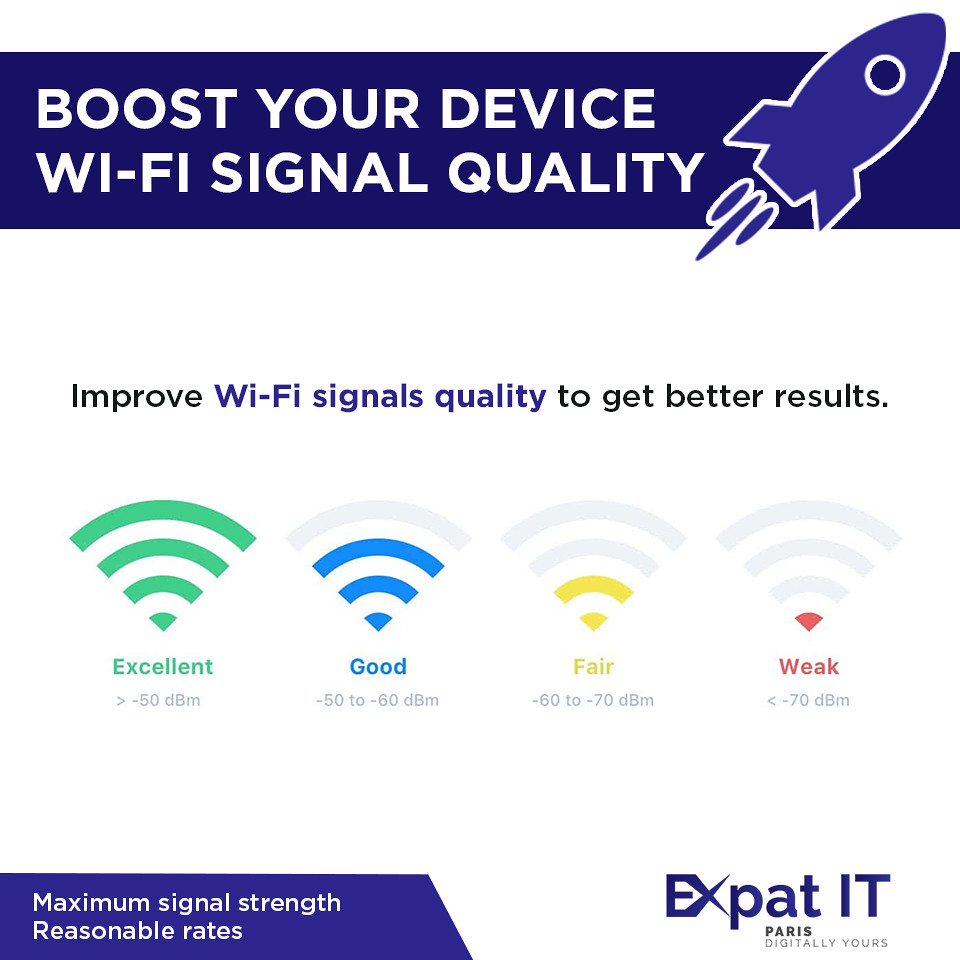The image features an advertisement for a Wi-Fi service with a clear, informational layout on a white background. At the top, a navy blue rectangular bar houses the white text "Boost Your Device Wi-Fi Signal Quality," accompanied by a blue rocket ship graphic shooting off the upper right-hand corner. Below this header, a detailed infographic displays Wi-Fi signal strengths from excellent to weak. The "Excellent" signal, in green, shows four bars at greater than -50 dBm. The "Good" signal, in blue, shows three bars ranging from -50 to -60 dBm. The "Fair" signal, in yellow, is represented by two bars within the -60 to -70 dBm range. The weakest signal, in red, shows a single bar at less than -70 dBm. At the bottom of the image, a small purple box with white text emphasizes "Maximum Signal Strength, Reasonable Rates." In the lower right-hand corner, the company name "Expat IT, Paris Digitally Yours" is featured, identifying the advertisement as a promotion for boosting Wi-Fi quality.